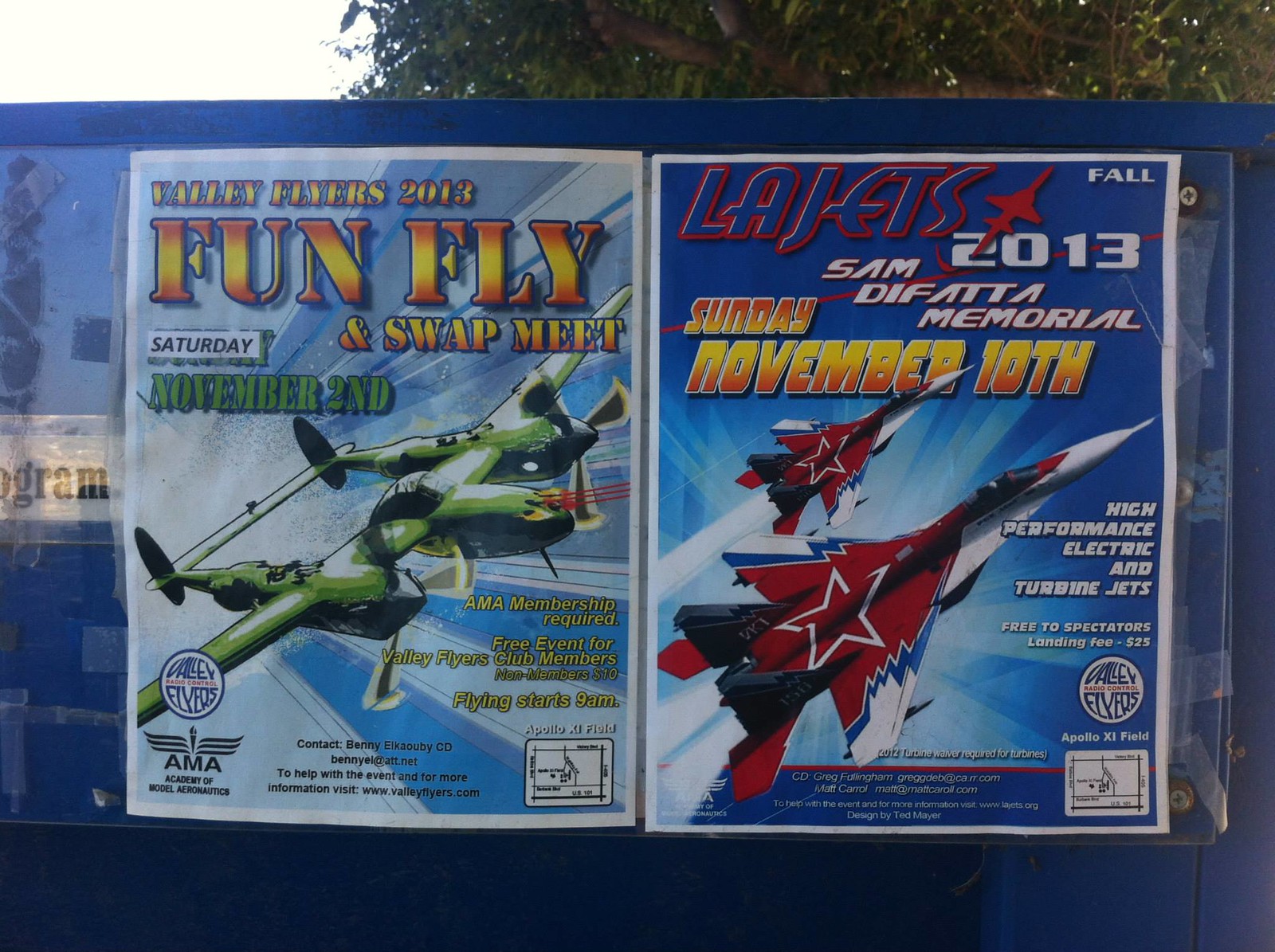The image is a wide rectangular shot of two large posters on a dark blue billboard. The top of the image reveals a green tree with dark brown branches against a white sky on the left. The poster on the left features a green, military-style plane flying diagonally to the right against a light blue background. It announces the "Valley Flyers 2013 Fun Fly and Swap Meet" in bold yellow and orange font with a bright dark blue border. Below that, it provides details: "Saturday, November 2nd, AMA membership required, free event for Valley Flyers Club members, non-members $10, flying starts at 9 AM at Apollo 11 field," along with contact information for Benny L. Cobby (BennyL at att.net) for further details.

To the right, a similar poster with a blue background showcases two red, white, and blue rockets with stars, heading towards the top right corner. This poster reads "LA Jets Fall 2013, Sam DeFatta Memorial, Sunday, November 10th," highlighting "high performance electric and turbine jets, free to spectators, landing fee $25," at the same Apollo 11 field. Contact details include Greg Fulingham (gregdeb at ca.rr.com) and Matt Carroll (mattatmattcarroll.com). The posters, designed to promote events organized by the Valley Flyers, also acknowledge Ted Meyer for the design. Above the posters, the sky and tree provide a contrasting natural backdrop to the vibrant and informative event announcements.